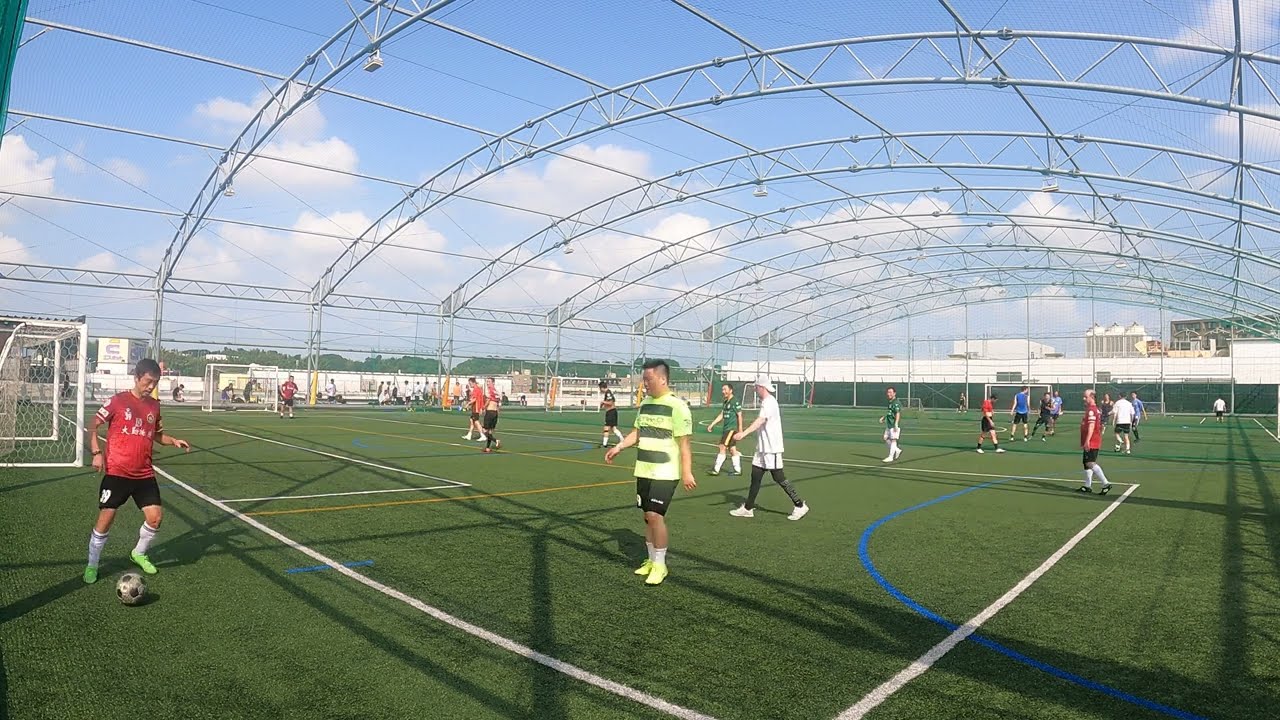The image captures an expansive outdoor soccer field with vibrant artificial green grass adorned with intricate white, yellow, and blue lines marking various play areas. Central to the scene is an ongoing casual soccer game featuring participants in mixed attire, though several players wear a uniform consisting of red shirts, black shorts, and neon green shoes. Notably, a player in red and black appears poised to kick a soccer ball, standing on one foot with the other mid-air, and sporting white socks.

To the left, the white-framed soccer net with white netting is visible. The scene is framed by a substantial metal structure above, which supports a retractable cover for weather protection and houses lighting fixtures for night games. The open framework also includes a net, allowing a view of the bright blue sky adorned with fluffy white clouds. In the distance, a large, long white industrial building can be seen, adding to the backdrop. This well-maintained field is part of a multi-field complex, as evidenced by the presence of multiple goals and the visible layout of three distinct soccer fields.